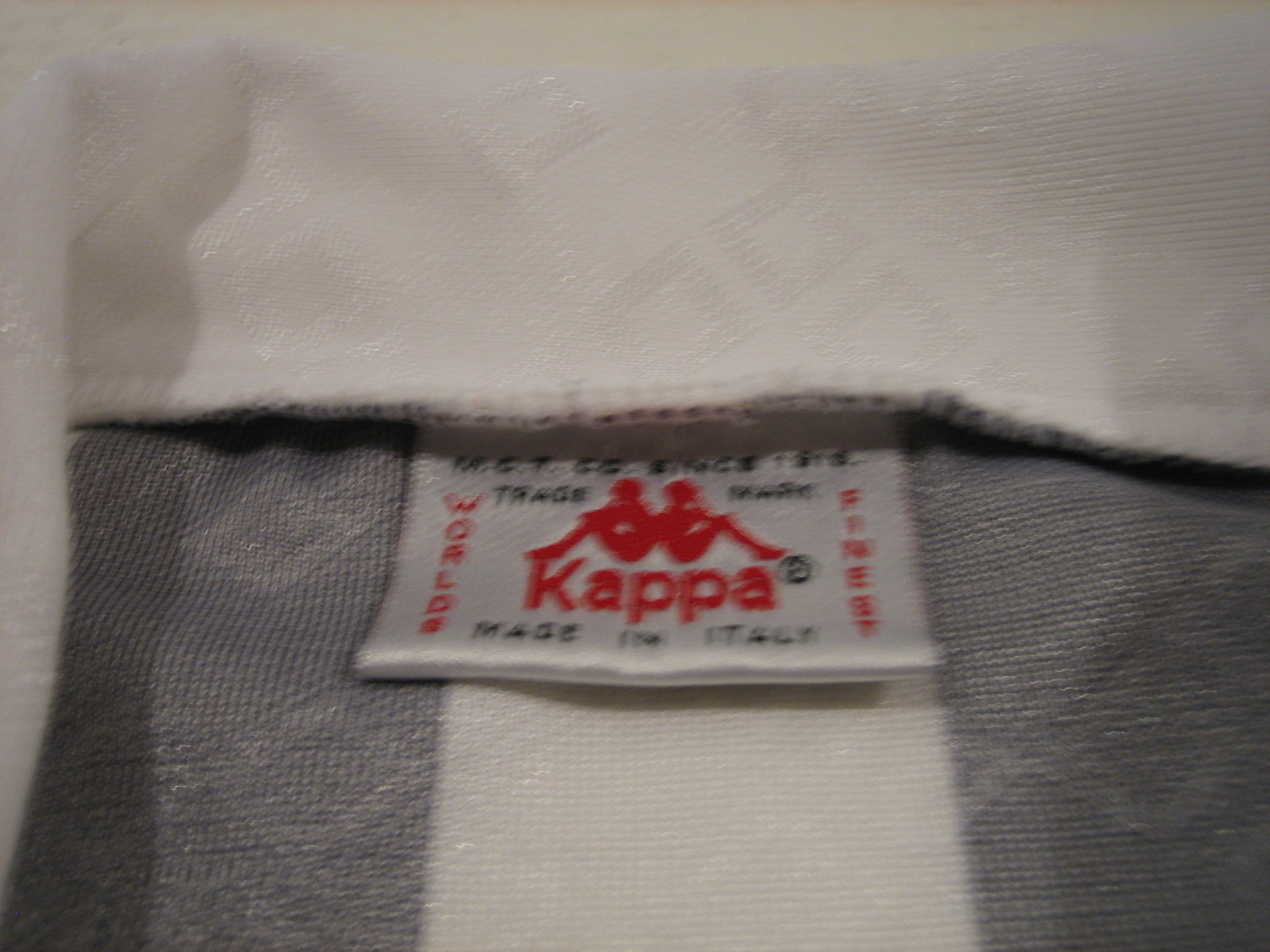This image displays a detailed close-up of a rectangular garment tag stitched inside a cloth shirt or possibly a bag, visible along the seam on the inside. The background fabric of the garment is a cream-colored cloth that transitions into a white-colored section adorned with a pattern comprised of square shapes in slightly darker tones. Below this are vertical stripes, alternating between gray and white, with a gray stripe followed by a white one, then gray again.

The tag itself is predominantly white with both black and red text along with a distinctive image. At the top, in black text, there are the letters "MGT" and additional words rendered indistinctly due to shadowing. The word "trade" is also visible in black. The centerpiece of the tag is emblazoned in red, featuring the word "Kappa" in large letters accompanied by an image of two individuals sitting back-to-back, one male and one female, executed in red as well. Below this image, the name "Kappa" is spelled out in capital letters. On the bottom in black text, the tag states "Made in Italy." Additionally, "World" is written vertically on the left side of the tag and "Finest" on the right, both in red text.

This comprehensive depiction highlights the tag's textual and visual elements while also detailing the fabric and pattern of the garment to which it is attached.